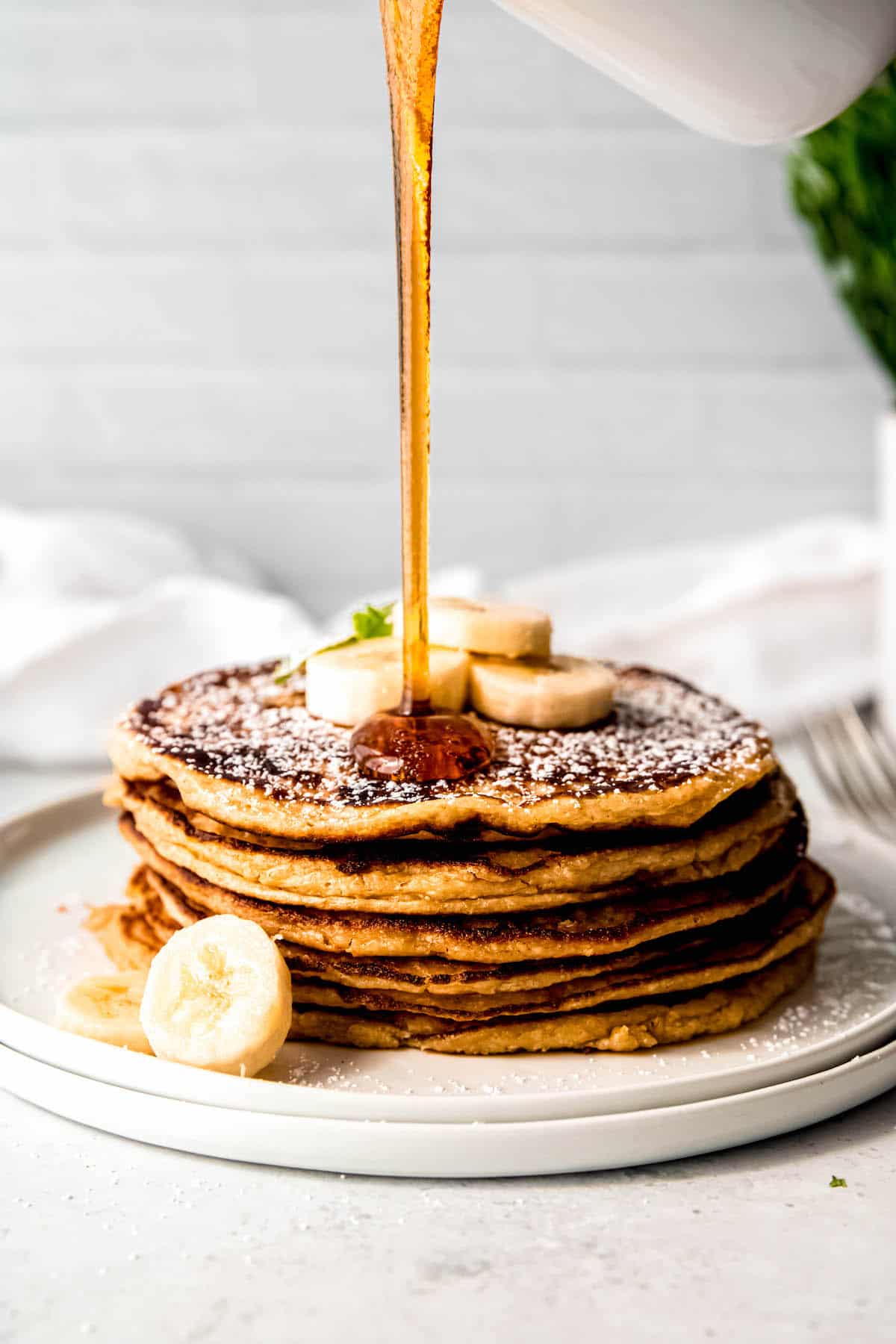This close-up photograph captures a delectable stack of golden-brown, crispy pancakes, dramatically drizzled with syrup pouring from an overhead white ceramic dish. The syrup cascades onto the top pancake, forming a glossy, enticing pool. Three thin banana slices and a sprinkle of powdered sugar embellish the topmost pancake, adding a touch of sweetness and texture. To the left side of the white plate, additional banana slices are artfully placed, alongside a sprig of green garnish. The plate itself rests on a pristine white marble table. In the softly blurred background, a white brick wall can be seen, subtly hinting at the cozy setting. Also slightly out of focus, a fork appears on the right, poised for the delicious undertaking.